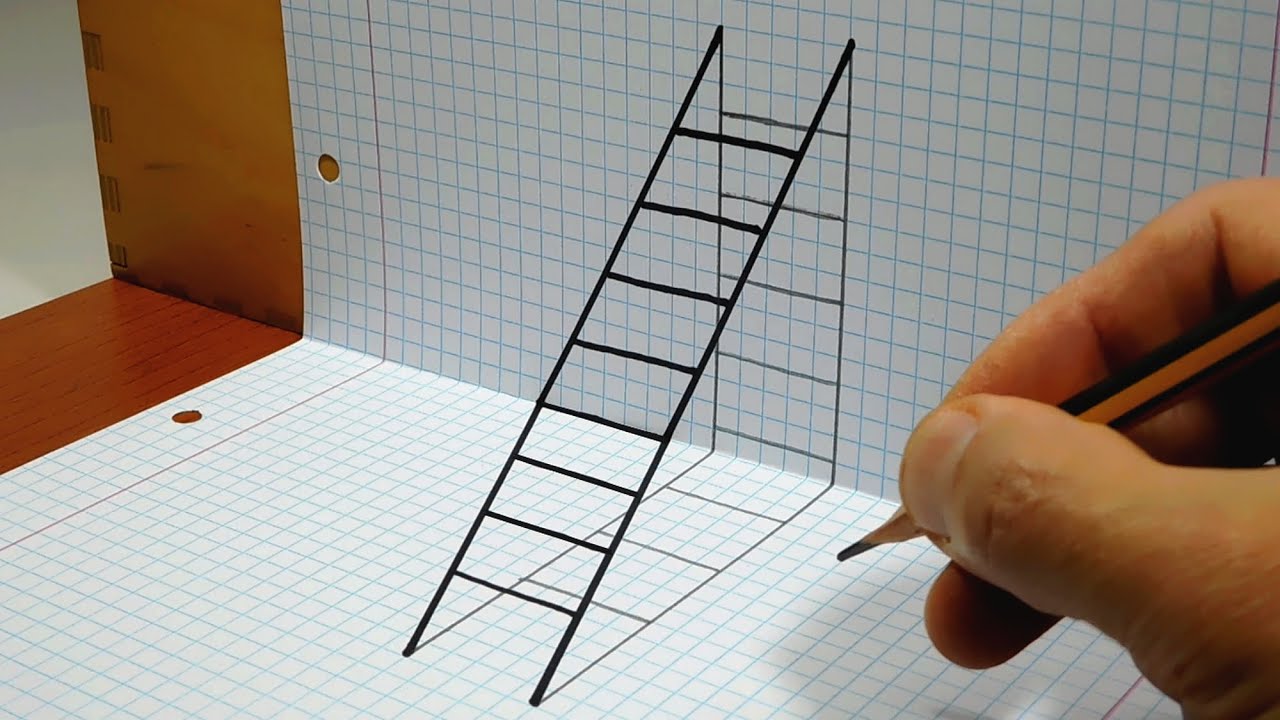In this artistic photo, a man's hand grips a standard orange Number 2 pencil as he meticulously draws an optical illusion of a ladder on a piece of white graph paper. The graph paper, covered in small squares, is partially folded, creating an effect that makes the ladder appear three-dimensional. The ladder, drawn in black with eight steps, seems to stand or lean against a wall due to the skilled shading and the paper's strategic bend. The precise shadowing alongside the folded paper enhances the illusion, making the ladder look authentic and three-dimensional to the viewer. The desk and wall are subtly visible in the background, further grounding the scene in reality.